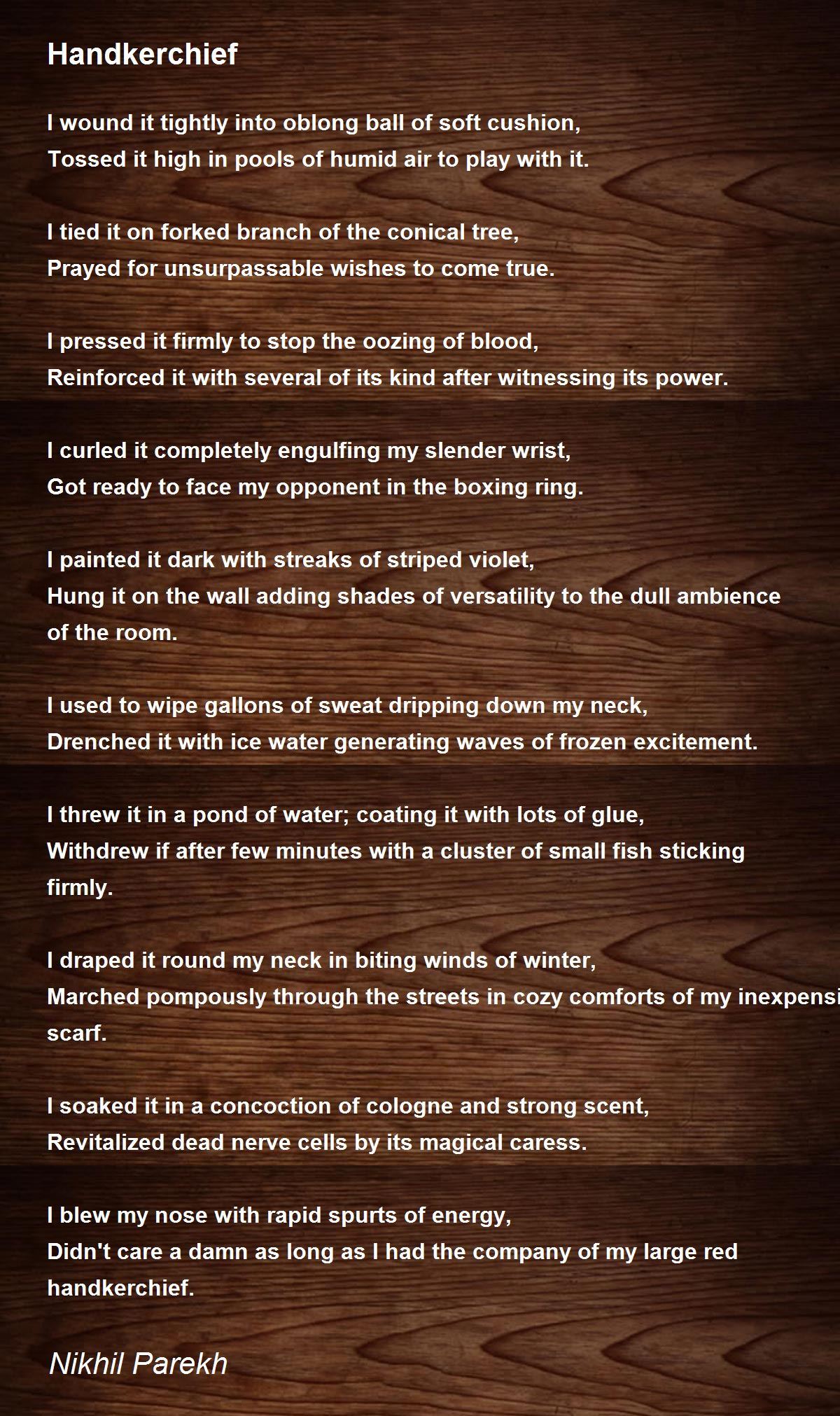The image features a horizontally oriented poem titled "Handkerchief" set against a brown wooden background with visible wood swirls. The poem, written in white text by Nikhil Parekh, begins with the repeated word "handkerchief" at the top, followed by a poignant narrative exploring various imaginative uses for a handkerchief. The verses weave through different scenarios: tightly winding the handkerchief into oblong balls of soft cushion and tossing it into humid air, tying it on a forked branch to pray for unsurpassable wishes, and pressing it to stop blood from oozing, reinforced by others of its kind. It continues with wrapping it around the wrist for a boxing match, painting it with violet streaks to embellish a room, using it to wipe sweat, soaking it in ice water for refreshment, throwing it in a pond to attract fish, draping it around the neck as a shield against winter winds, soaking it in cologne, and finally using it to blow the nose with defiant vigor. The poem ends with the poet's name, Nikhil Parekh, at the bottom in white font.